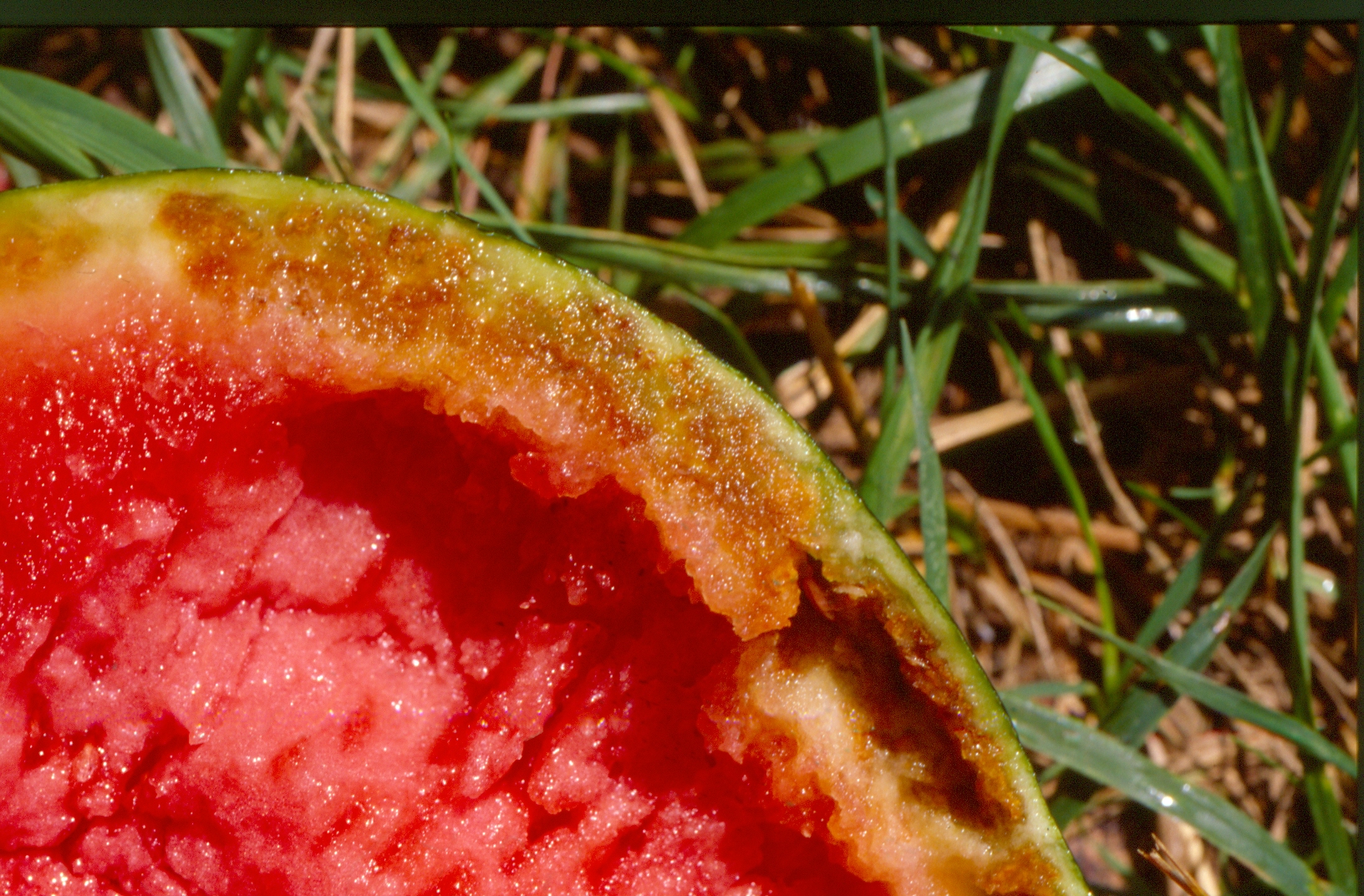This image is a color photograph featuring a discarded piece of fruit, possibly a watermelon, lying on a bed of green and brown, partially dried grass. The fruit, situated primarily in the bottom left part of the photo, appears to have been split open, revealing its vibrant pink flesh. The outer rind of the fruit is green, transitioning to white with brown spots indicative of rotting. The fruit has clearly been exposed to the sun for some time, as highlighted by the stark contrast between the bright, juicy interior and the deteriorating outer layers. The photograph contains no people, animals, text, structures, or mechanical objects, focusing solely on the fruit and its immediate grassy surroundings.